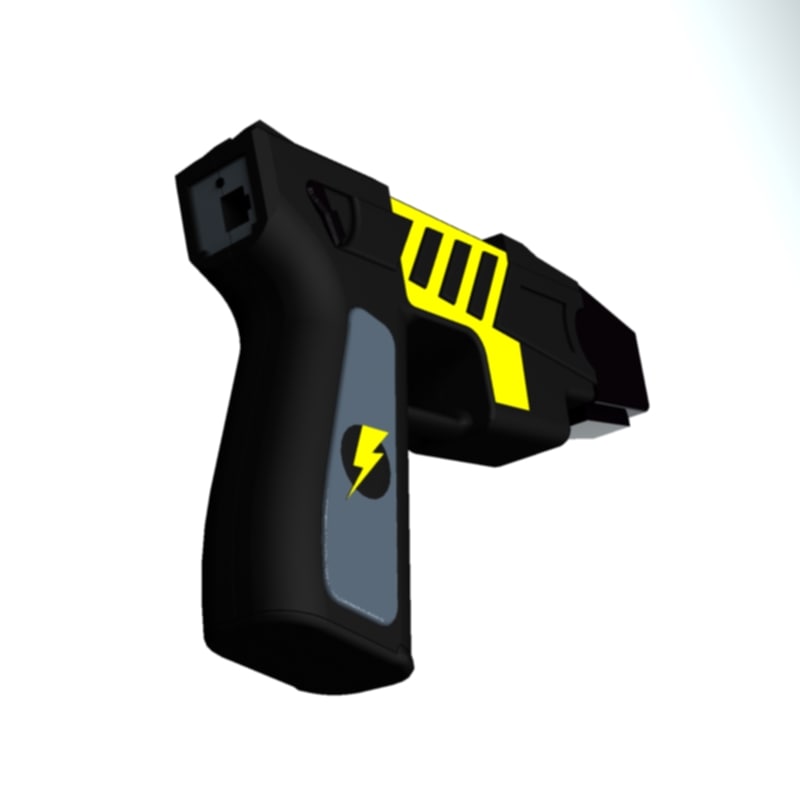The image depicts a highly detailed, digitally created drawing of a mechanical gun, focusing centrally within a square background that transitions from dark gray along the edges to white towards the center. The gun itself is black with prominent yellow accents, including a yellow lightning bolt on a black circle situated on the gray grip area. The handle features a hole resembling a USB port at the back. The design is angled diagonally with the barrel pointing towards the right, exposing both the side and bottom of the handle. The overall aesthetic of the gun is blocky and squared, with the yellow detailing extending towards the trigger area, giving it a distinctive look within the zoomed-in composition. There is no text or additional elements within the predominantly white and gray background, emphasizing the gun as the sole focus of the image.